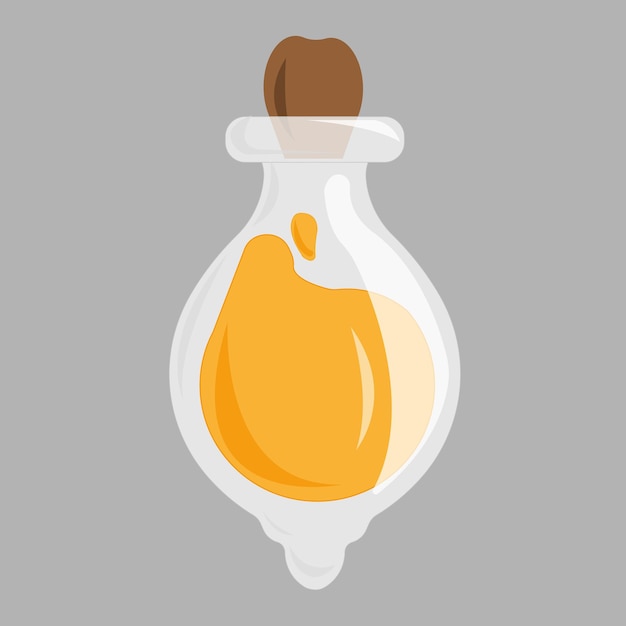This is a simplistic, cartoon-like illustration featuring a clear apothecary-style glass bottle against a flat gray background. The bottle has a round, almost tear-shaped bottom that narrows to a small neck at the top and is sealed with a brown cork stopper. The interior contains a smooth, yellow liquid reminiscent of honey. The shading on the bottle is minimal, providing just enough detail to suggest its roundness and the reflective nature of the glass. The liquid inside sits uniformly, adding to the overall clean and straightforward aesthetic of the image.